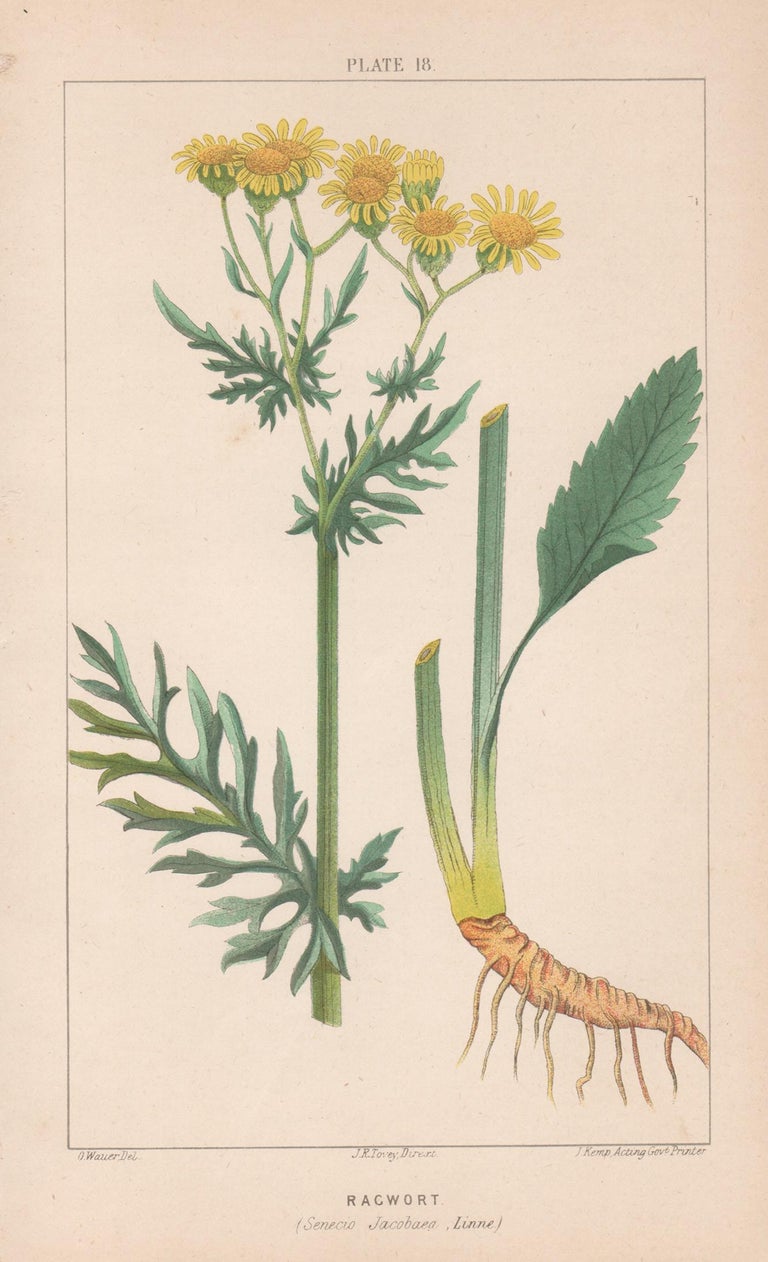The image is a scanned illustration of ragwort, resembling a scientific diagram you'd find in a textbook. The card features the label "PLATE 18" in uppercase gray letters at the top, with the word "RAGWORT" in gray at the bottom, accompanied by some other small, illegible text. The image shows a detailed depiction of a ragwort plant with a long green stalk that branches into smaller stalks, each ending in a yellow flower with sunflower-like petals and darker yellow to almost orange centers. At the top of the illustration, there is a prominent green leaf with finger-like divisions, while smaller leaves appear further up the stalk. The root system, portrayed in detail on the right side of the card, reveals a main taproot with several smaller roots extending from it. The card itself has a thin, light gray frame and is printed on an off-white, almost peach-colored paper.